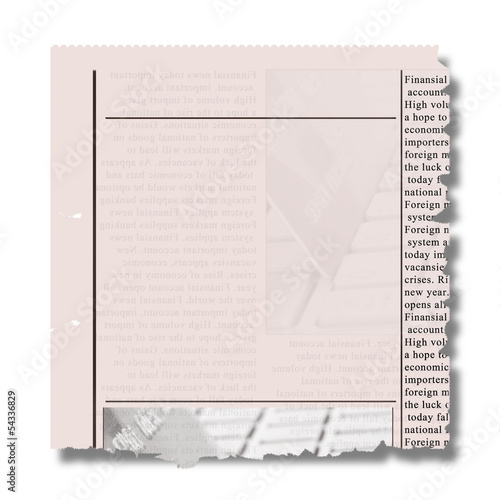This Adobe stock image, identified by the number 54336829, depicts a torn corner of a newspaper page with a distinctive blank square at its center, bordered by black lines, likely indicative of a space reserved for an ad or other content. The left edge is straight while the top shows a small scalloped edge and both the bottom and right sides are ragged as if ripped away from the main newspaper. Along the left side, a thick vertical line is present, with Adobe stock watermarks diagonally spanning across the image. Additionally, hints of text and a photo from the torn part of the newspaper are visible at the edges, with partial words such as "financial," "account," "high volume," and "foreign" discernable in the obscured print. The background paper has a slight tint of red, pink, or perhaps orange, highlighting the transparency typical of newsprint, revealing faint images and text from the reverse side.